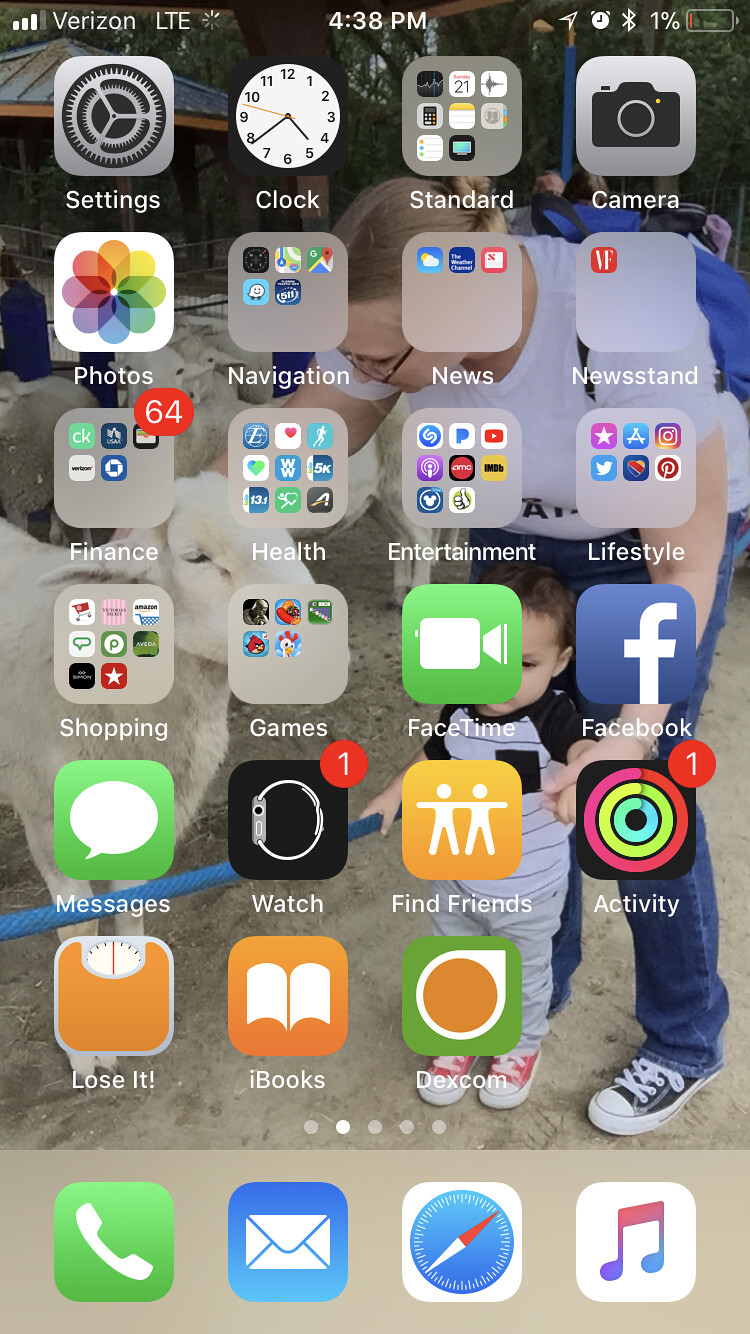The image depicts the home screen of an iPhone, with Verizon as the service provider, displaying the time as 4:38 PM. The phone's Bluetooth is activated, and the battery level is critically low at 1%. The screen features a standard array of applications and folders. Visible apps include Settings, Clock, Camera, and Photos. Several categorized folders are present: Navigation, News, Finance, Health, Entertainment, Lifestyle, and Games. The Lifestyle folder contains social media apps like Twitter, Instagram, and Pinterest. Notably, there are standalone apps for Facebook and FaceTime, affirming the device is an iPhone. Notifications are visible for the Watch App and Activity App. Additionally, the home screen includes the Find Friends app and the Books app.